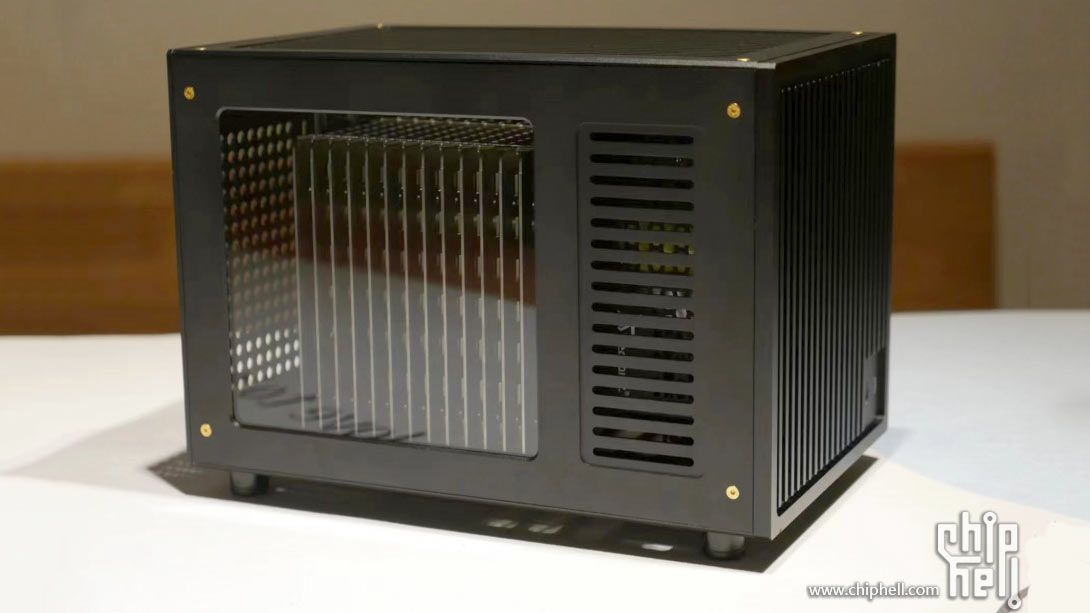This color photograph, set against a beige background, serves as an advertisement for a product featured on www.chiphell.com. Central to the image is a black metallic box placed prominently on a pristine white table. The box, which suggests the appearance of either a heater or a part of a computer, is equipped with small black feet for stability. The sides of the box feature an array of vents: large grill-like apertures facilitate air flow while the front sports a smaller grating area adorned with four gold screws in each corner, which accentuate its industrial aesthetic. The interior, visible through a glass window on the front, reveals metal bars or a layered apparatus that hints at its functional purpose, possibly for heating or electronic use. In the background, a wooden bench or the back of a chair provides context and adds a touch of casual ambiance to the setting. The lower right corner of the image is branded with a logo that includes the website address www.chiphell.com, subtly directing viewers to further information.